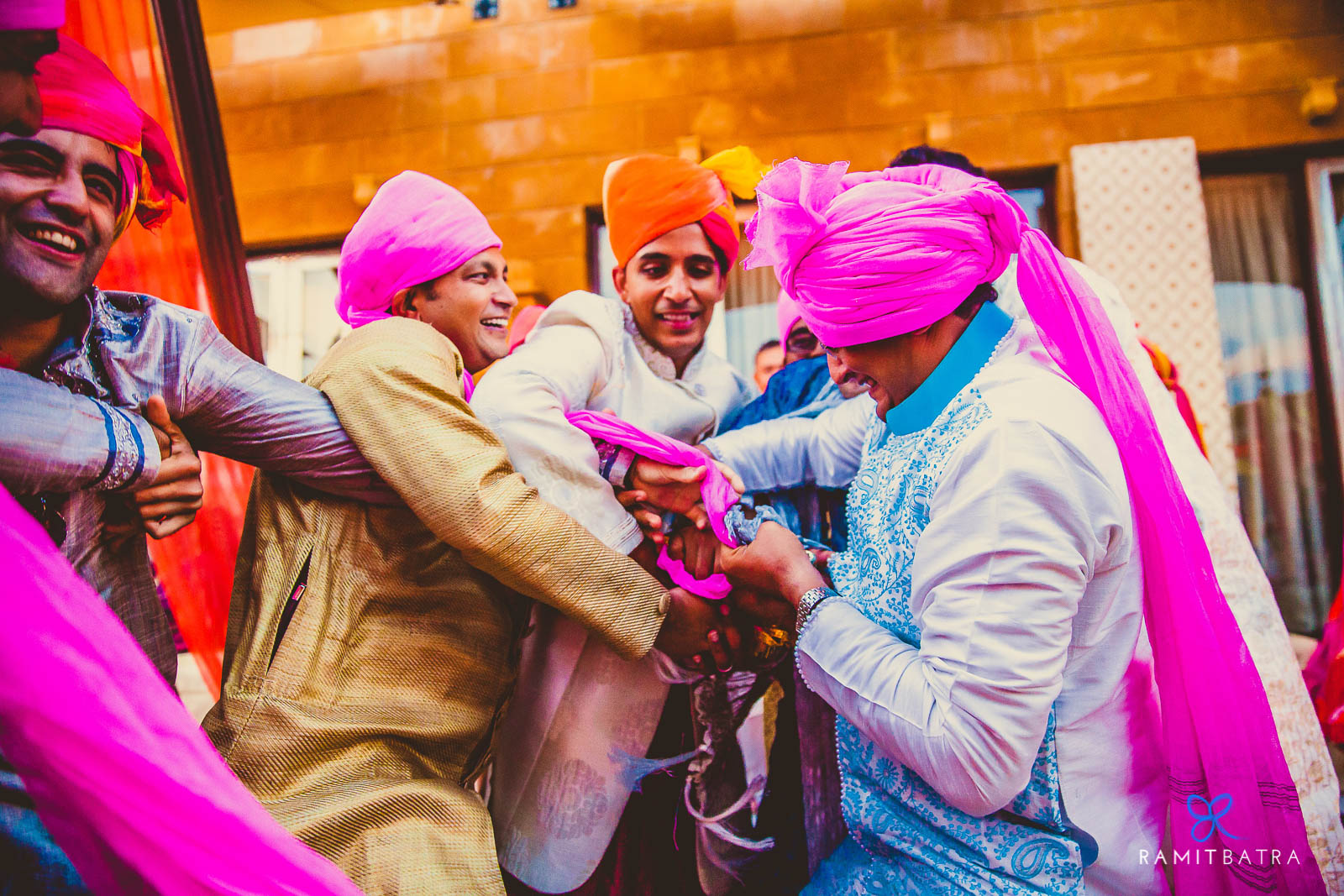The image depicts a group of four to five men who appear to be of Middle Eastern or Indian descent, wearing vibrant traditional attire. They are engaged in a central handshake or perhaps struggling to hold onto a piece of fabric, indicating a possible cultural or ceremonial activity. The men are adorned in bright colors including pinks, oranges, blues, yellows, and whites, with headdresses, turbans, and scarves adding to the vivid display. The man on the right side stands out in a long pink headdress extending down his back, paired with a blue-accented cassock. He is shaking hands with another man in an orange turban and a white coat. Adjacent to them, another man with a pink headdress and a brown coat is also visible. The background features an orange building, and in the bottom right corner of the photo, the text "Ramit Batra" is evident, suggesting the possibility of Indian customs or an Indian wedding. The left corner of the photo shows several other men contributing to the handshake or fabric-holding gesture, enhancing the communal aspect of the scene.